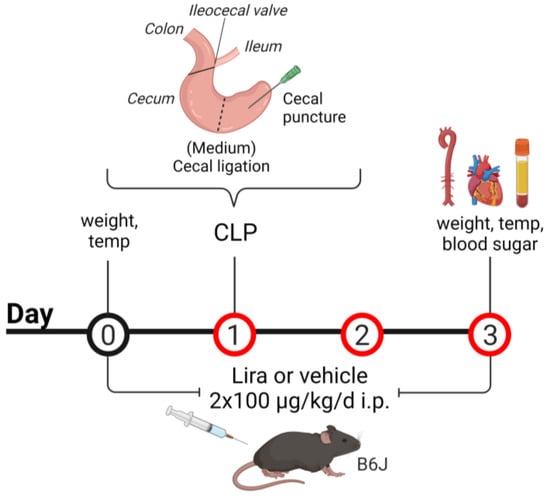The image is a detailed diagram likely illustrating a scientific experiment related to the impact of food consumption and energy on a rat, possibly designed for educational purposes such as a textbook or a presentation. At the top of the diagram, there is a pink illustration of a stomach labeled with various parts: colon, ileocecal valve, ileum, cecum, medium cecal ligation, and cecal puncture. Below the stomach, "CLP" (abbreviated for Cecal Ligation and Puncture) is prominently noted, directing attention through a series of numbered and colored circles (1, 2, and 3) which are possibly indicative of different experimental days or steps in the process (Day 0, Day 1, Day 2, Day 3). 

To the right of the diagram, a black line extends from zero marked with parameters such as weight, temperature, and blood sugar. This line connects to an illustration of a rat labeled "B6J", accompanied by a syringe. Notations such as "lira or vehicle, 2 times 100" further expand details of the experiment. Additional lines detail measurement points such as weight, temperature, and blood sugar, which are also associated with visual representations of a heart and a vial of blood. This comprehensive illustration encapsulates various stages and variables critical to the experimental setup, providing a clear and detailed visual guide.